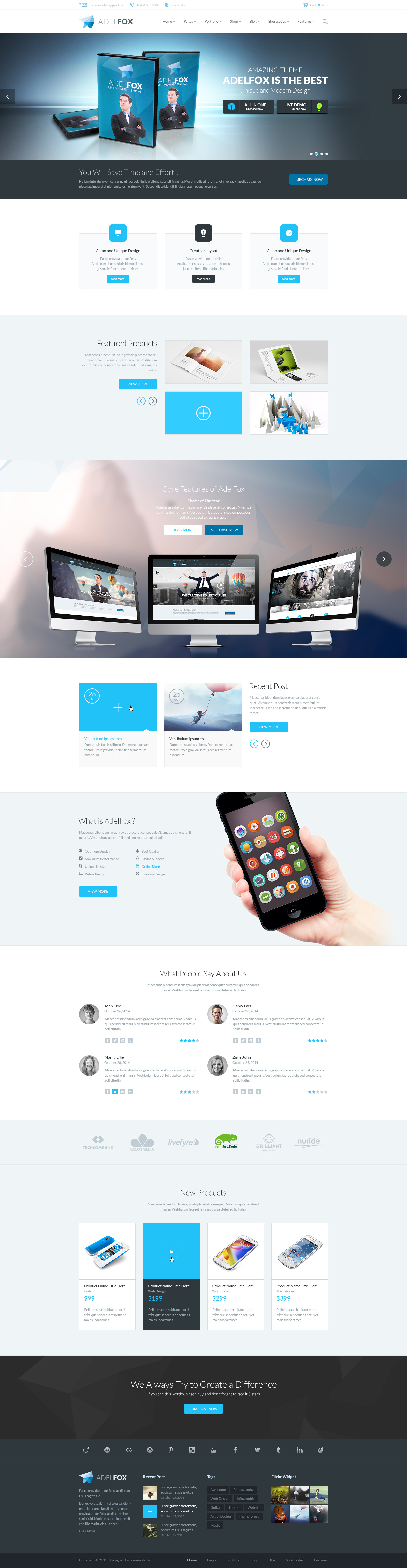The screenshot showcases an informational app with a cluttered interface and very small, unreadable text. At the top, there is a rectangular image featuring three DVDs. Below it, a series of light gray tiles with various buttons are displayed. One specific tile contains six small images. Further down, a larger tile prominently features an image of three flat-screen monitors. Underneath this, there’s a picture of a hand holding a smartphone. Below the smartphone image, four snippets of text are visible, but they are too small to be decipherable. The last section of the interface consists of another light gray tile with four sub-menus displayed in white, potentially related to smartphones or some form of technology, indicating that this is an informational page online.